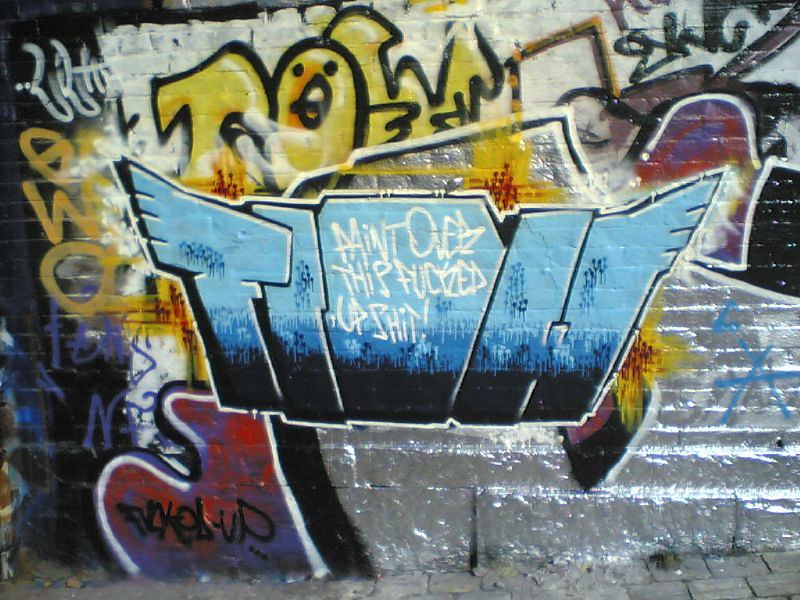This is a horizontally aligned rectangular image depicting a vibrant graffiti mural on the side of a brick wall, likely in an urban alleyway or city setting. The bottom edge of the image features a portion of the stone-brick sidewalk. The graffiti is a colorful blend of blue, black, yellow, silver, and hints of purplish-maroon, with some white highlights. At the center of the mural, blue and black spray paint forms an abstract shape that resembles wings but lacks a discernible bird's face. This section includes white text that reads, "paint this fugged up shit I guess." Above or behind this, additional graffiti features the letters "EWO" on the left side and the outline of a yellow bird with black dots for eyes and a black circle for a beak. The lower right-hand corner reveals a segment of the wall where silver paint overlays the brick surface. The mural appears to be the work of multiple artists, layering and covering pieces of each other's art.